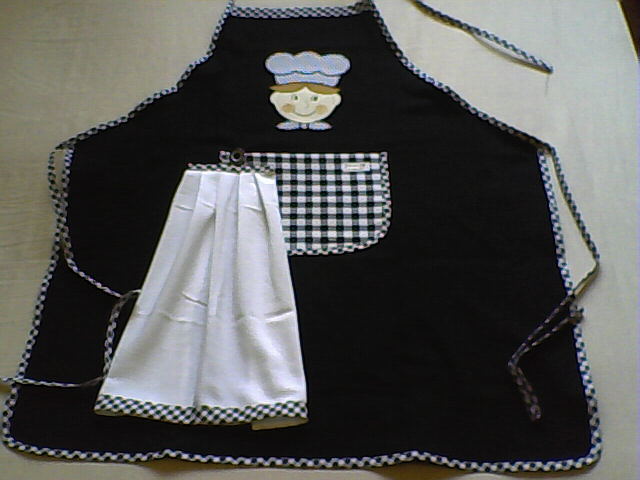This image features a black apron laid neatly on an off-white surface. The apron is adorned with an eye-catching black and white checkered print edging, which also extends to the straps. At the center, there is a prominent black and white checkered pocket. Above this pocket, a white linen cloth with pleated folds and the same checkered border peeks out, adding an element of texture and contrast. Dominating the upper section of the apron is an appliqué or patch depicting a cheerful cartoon chef. The chef has brown hair slightly winged out from under a short gray chef's hat and wears a gray bow tie. His face is animated with rosy cheeks and a broad smile, bringing a playful touch to the design. The overall image portrays a stylish yet functional kitchen apron with intricate detailing and a whimsical chef illustration.